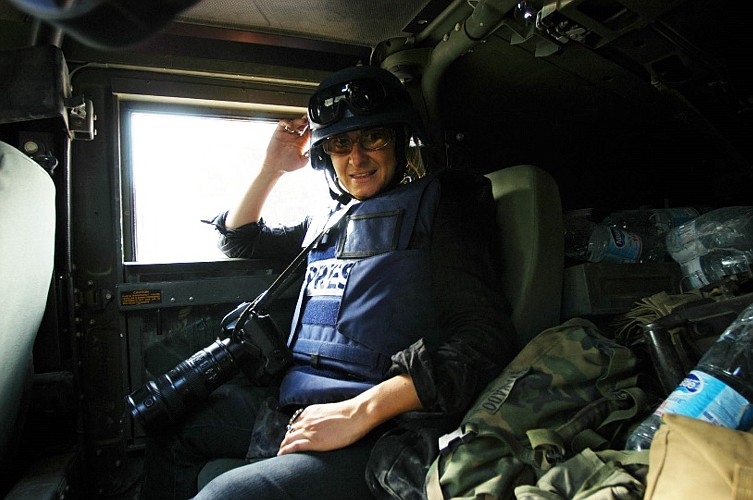The photo depicts the interior of a vehicle, likely a helicopter or possibly a Humvee, on an army base in a war zone circa the late 90s or early 2000s. The focal point is a photographer seated in a compact compartment, clad in a navy blue bulletproof vest labeled "Press." He is equipped with a large camera suited for journalism, featuring an intense zoom lens, which lays across his lap. The photographer is protected by a helmet while wearing sunglasses, with additional goggles resting atop his helmet. To his side is a camouflage duffel bag or jacket marked with a soldier's name, accompanied by numerous empty Nestle water bottles piled behind him. The window of the vehicle does not provide any discernible scenery, emphasizing the cramped and utilitarian nature of the setting.